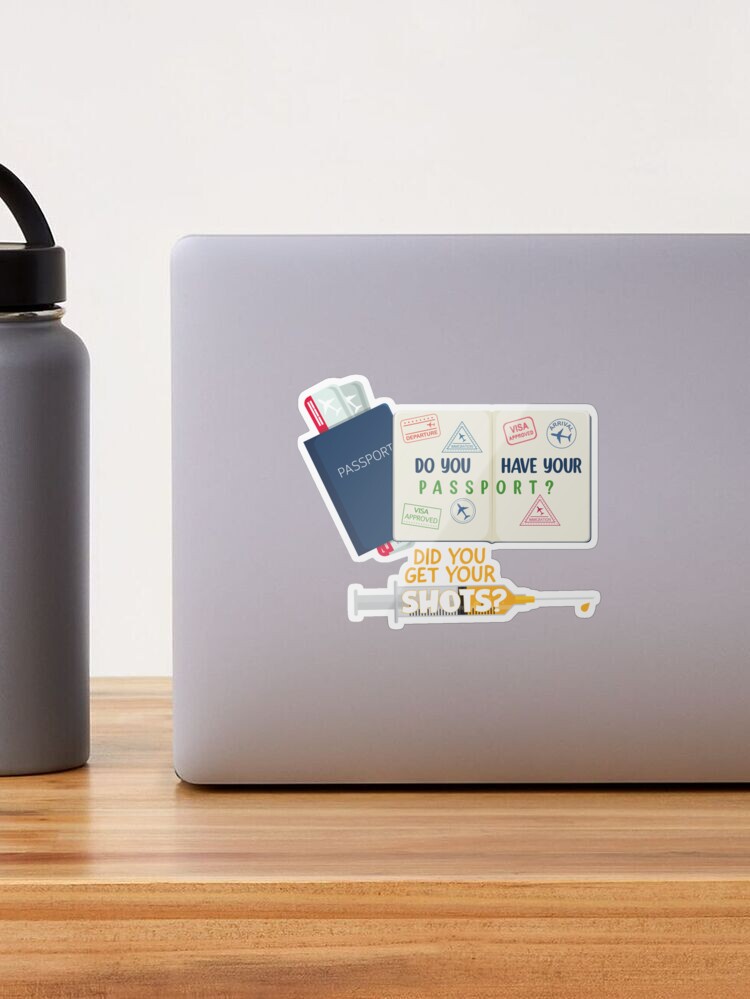In this detailed photograph, a light gray laptop is prominently featured with several distinct stickers adorning its top surface. The largest sticker depicts a closed blue passport with grey and red boarding passes protruding from it. Another sticker slightly overlaps, displaying an open passport with colorful stamps and the text "Do you have your passport?" in blue and green letters. Near these, a sticker of a syringe with yellow liquid dripping from the needle poses the question, "Did you get your shots?" in a mix of yellow and white text. Sitting adjacent to the laptop is a gray stainless steel water bottle with a black, screw-on lid, resembling a Hydro Flask design. Both the laptop and the bottle rest on a very light-colored wooden table, set against a plain white background.